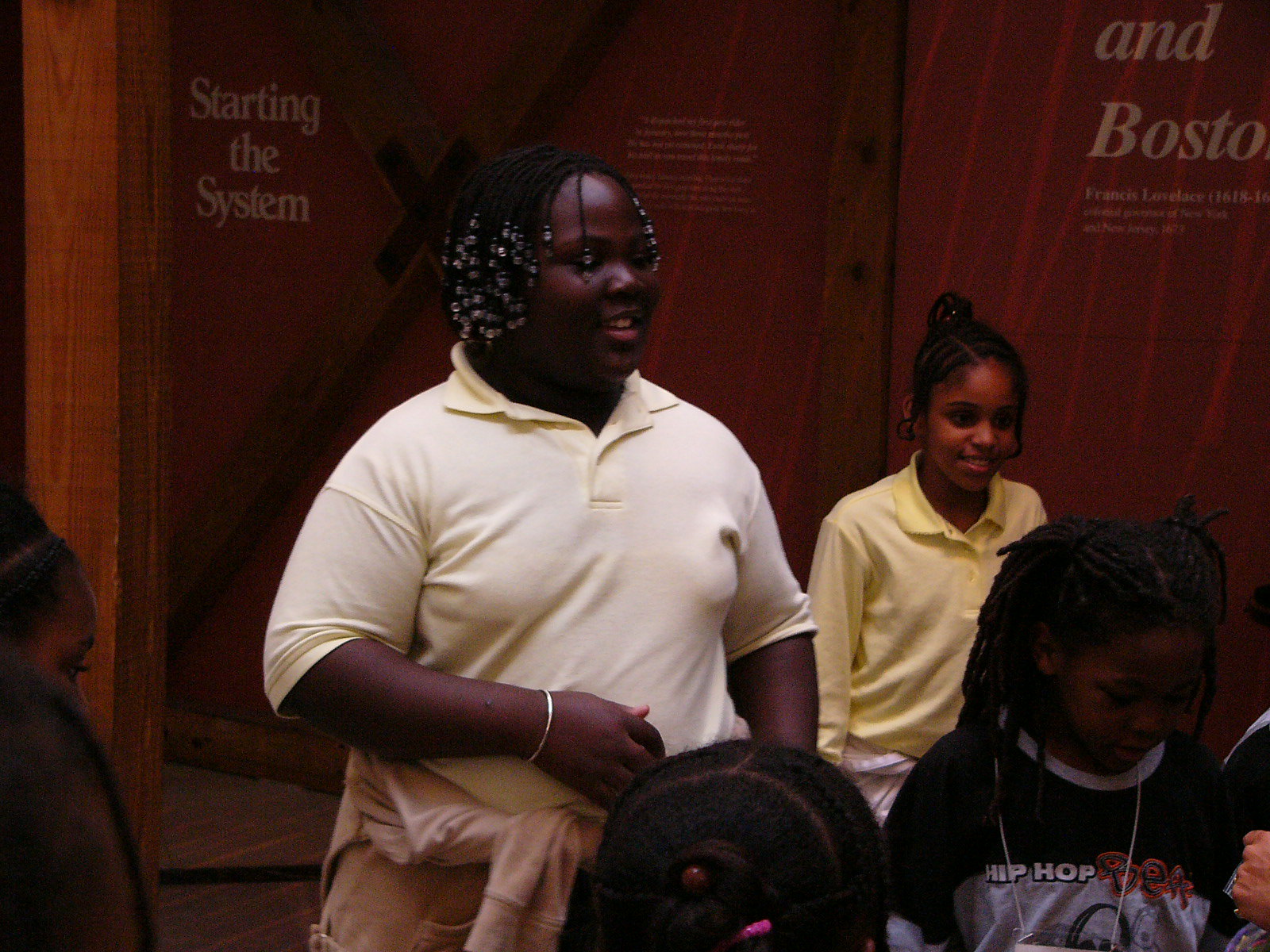The image depicts a group of elementary school-aged children, likely on a museum field trip. At the center, an African American girl wearing a pale yellow polo shirt stands out. She is slightly overweight, with braided hair adorned with beads extending to her chin, a sweater tied around her waist, and a bracelet on her right wrist. Beside her to the left, another girl in a yellow collared shirt and braided hair pulled back in a bun is visible. Both are framed against a wood-paneled wall with text that reads, "starting the system," and "and Boston," with the name "Francis Lovelace, 1618" beneath the word Boston. In the foreground, to the bottom right, a child in a black t-shirt with "hip hop poet" printed on it is seen. The overall setting is an indoor museum environment bustling with the children's excitement.